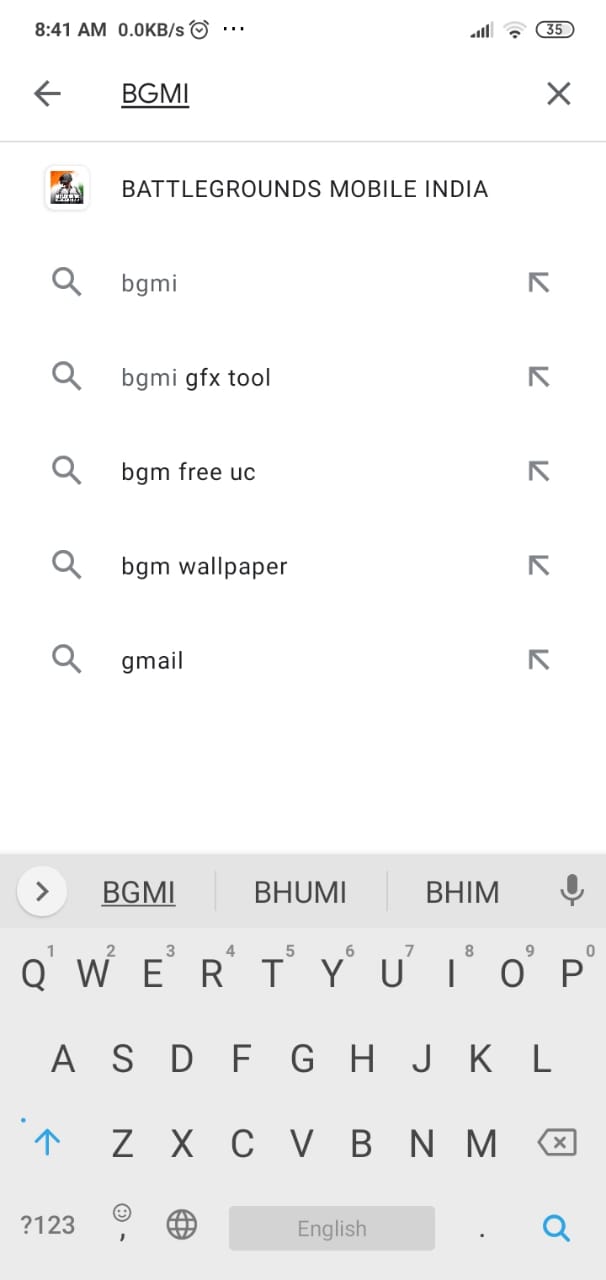This image is a screenshot of a web page taken at 8:41 a.m. as displayed in black letters at the top. To the right of the time, it shows "0.0 KB/s" followed by a clock icon and three vertical dots on the far-right side. Additionally, signal strength indicators for Wi-Fi are visible along with a small pill-like icon displaying the number three.

Just below this top bar, there's a navigation section with a left-pointing arrow and the letters "BGMI" in all caps and underlined. On the right side of this section, there's an "X" icon. Below this navigation line, a text label reads "Battlegrounds Mobile India."

Underneath this label is a list of search topics, each accompanied by a search icon. The first topic is "BGMI," followed by "BGMI GFX," "BGMI free," "BGMI wallpaper," and "Gmail." Beneath this list is a keyboard screen with predictive text suggestions at the top. These suggestions include "BGMI," "BH," "YOU," "MY," "BEACH," and "I AM," with an arrow pointing to the right within a circle icon. There is also a microphone icon beside the suggestions.

At the bottom of the screenshot is a standard QWERTY keyboard with no visible numbers, except for a button at the bottom left corner labeled "?123."